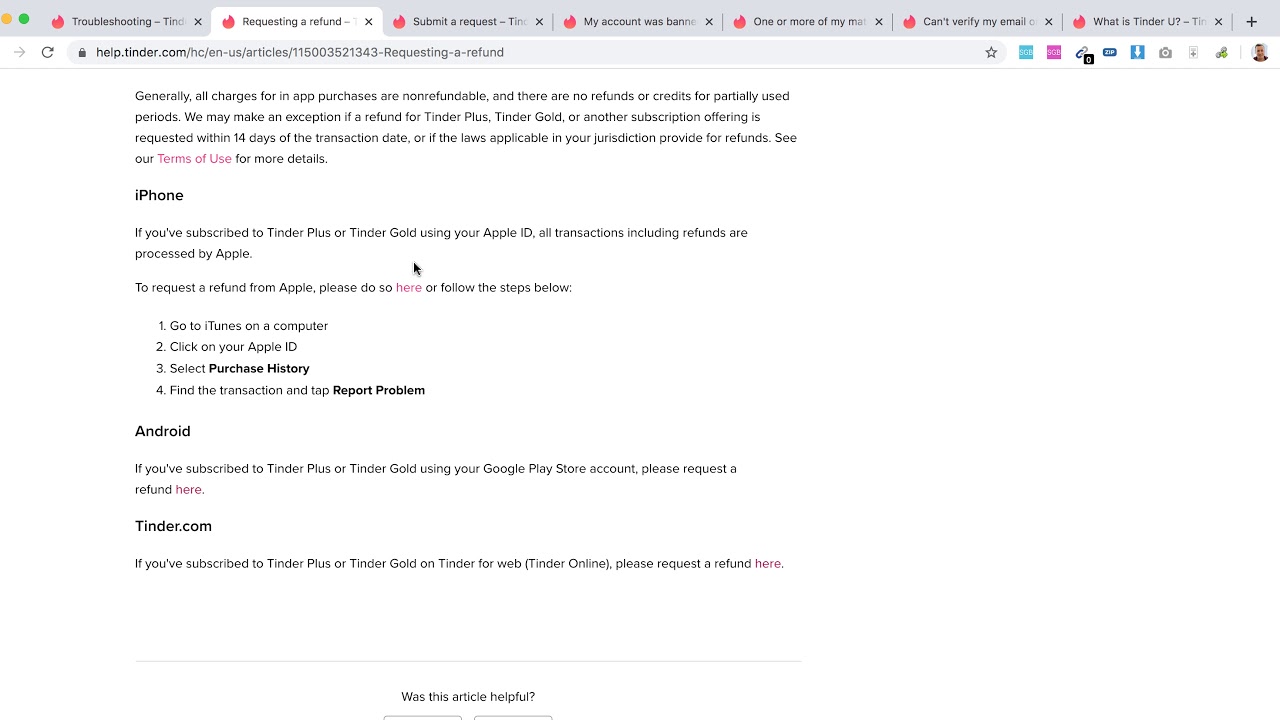The image depicts a desktop application displaying the Safari browser interface. The main focus is on a second tab labeled "Requesting a Refund" within the browser, which is currently active. Adjacent tabs, from left to right, include "Troubleshooting Tinder," "Submit a Request," "My Account Was Banned," "One or More of My...," "Can't Verify My Email," and "What is Tinder U?" 

The URL shown for the active tab is detailed as “help.tinder.com/hc/en-us/articles/115003521343-requesting-a-refund.” A star symbol, located to the right of the URL, presumably allows users to bookmark the page.

The content of the page primarily details Tinder’s refund policy. It states that generally, charges for in-app purchases—including Tinder Plus, Tinder Gold, or similar subscription services—are non-refundable, and no credits are offered for partially used periods. However, it mentions an exception for refunds requested within 14 days of the transaction date, or as provided by applicable laws. A hyperlink with a slightly pinkish hue directs users to the "Terms of Use" for more detailed information.

Further explanations are available for refund requests specific to iPhone, Android, and tinder.com platforms. At the bottom of the screenshot, users are prompted with the question, "Was this article helpful?"